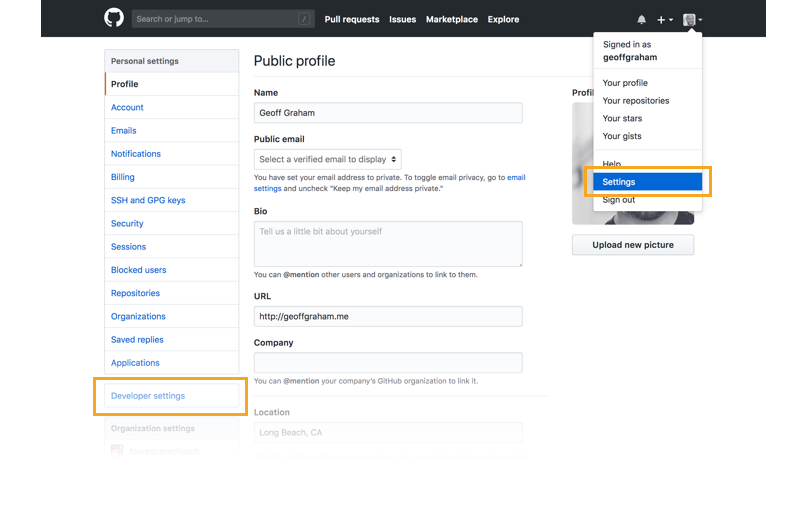The image depicts a user interface on a white background. At the top of the image, there is a long black navigation bar. On the left side of this bar, there's a circular icon resembling a cat's head, which is followed by a search box. Further along the bar, there are labeled tabs: "Pull requests," "Issues," "Marketplace," and "Explore." Toward the right side of the navigation bar, there is a bell icon, a plus sign, a down arrow, and a tiny square with an image inside it.

Clicking on the tiny square reveals a dropdown menu that includes the following options: "Signed in as Jeff Graham," "Your profile," "Your repositories," "Your stars," "Your gists," "Help," and "Settings." The "Settings" option is highlighted with a yellow block around it. Beneath these options, there is a "Sign out" button.

On the left side of the main interface, there's a larger blue box at the top labeled "Personal settings." Below this box, a vertical menu on a white background with a small red line includes items such as "Profile" in black text. In blue text, it lists "Account," "Emails," "Notifications," "Billing," "Shipping and Handling," "GPG Keys," "Security Sessions," "Blocked Users," "Repositories," "Organizations," "Saved Replies," and "Applications." An orange box highlights the "Developer settings" item in this menu.

On the right side of the interface, there is a section labeled "Public profile" with various fields. These fields include "Name," filled in with "Jeff Graham," and "Public email," which allows selection of a verified email through an up and down button. Following these are fields for "Bio" with an accompanying text box, "URL" with an HTTP address provided, and "Company." There is an additional line for "Location."

Finally, beneath the dropdown menu labeled "Signed in as Jeff Graham," there is an option to "Upload new picture," and Jeff's old picture is displayed below this option.